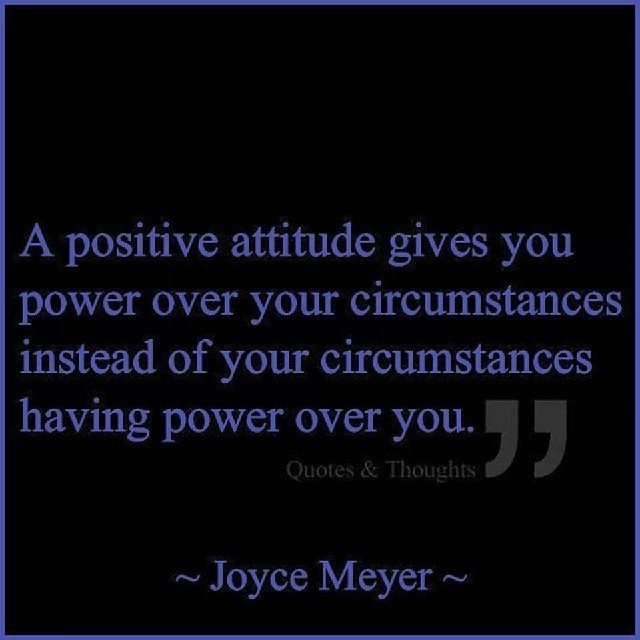The image features a large black square background with a bluish-purple border. Centered within the square is an inspirational quote in a bluish-purple font that reads, "A positive attitude gives you power over your circumstances instead of your circumstances having power over you." The quote is attributed to Joyce Meyer, with her name placed prominently at the bottom of the square in the same bluish-purple color. At the end of the quote, there are large gray quotation marks, followed by the words "Quotes and Thoughts" in a gray font, reinforcing the theme of positive thinking.